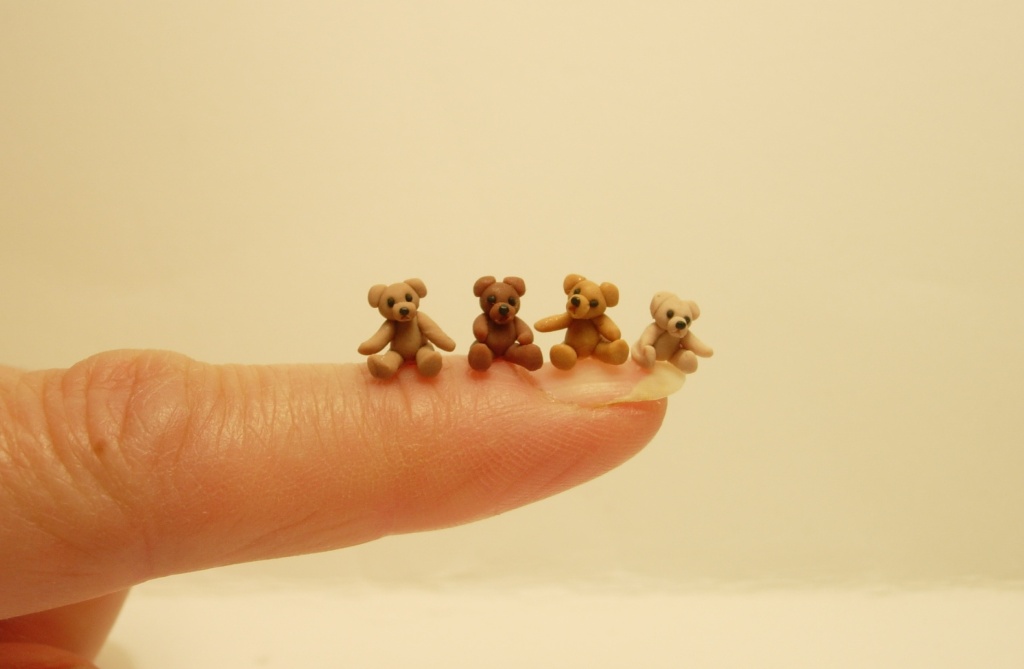In this close-up photograph, we see a person's left index finger extended from the bottom left into the frame, set against a plain, cream-colored background, likely cardstock or paper. Resting atop the fingertip are four tiny, cartoony clay bears, each sitting in a row. From left to right, the colors of the bears are a beige-ish brown, dark brown, rich brown, and light brown. Each bear features a round head with round ears, a black dot for a nose, and two black dot eyes. The first two bears sit directly on the fingernail, with the second bear's leg slightly off the nail; the last two sit on the top of the finger. The first bear has an arm reaching slightly to the right, the second, in cinnamon color, has an arm stretching to the left, the third, the darkest bear, has bent arms, and the fourth, the lightest close to the hand, has both arms spread out. This delicate arrangement emphasizes the intricate and charming details of the bears, along with the gentle curve and detailed fingernail of the finger they sit on.